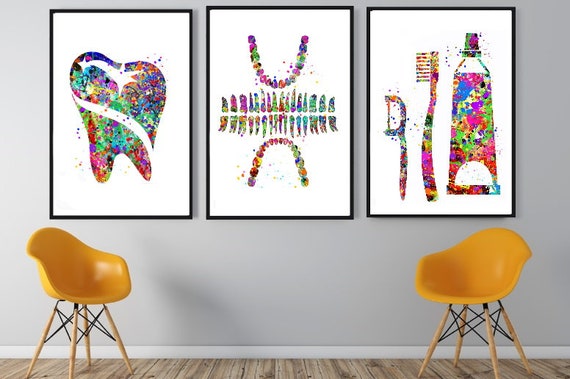This indoor scene features a contemporary setup with two vibrant yellow plastic chairs, notable for their small brown dowel legs crisscrossed with thick black cord for added stability. The chairs sit on a blondish wooden floor, against a gray wall accented with a thin white baseboard. Above the chairs, three vivid and colorful pieces of wall art, all related to dental care, add a playful touch to the setting. 

The left artwork features a large tooth shape adorned with splattered, multicolored patterns. The middle piece showcases upper and lower teeth impressions, rendered in the same lively, rainbow-hued splatters. The right-most art piece displays a detailed array of dental tools—a tooth flosser, a toothbrush, and a toothpaste tube, all brightly colored and positioned against the neutral backdrop. This triptych of multicolored dental images creates a dynamic contrast with the otherwise minimalist decor.